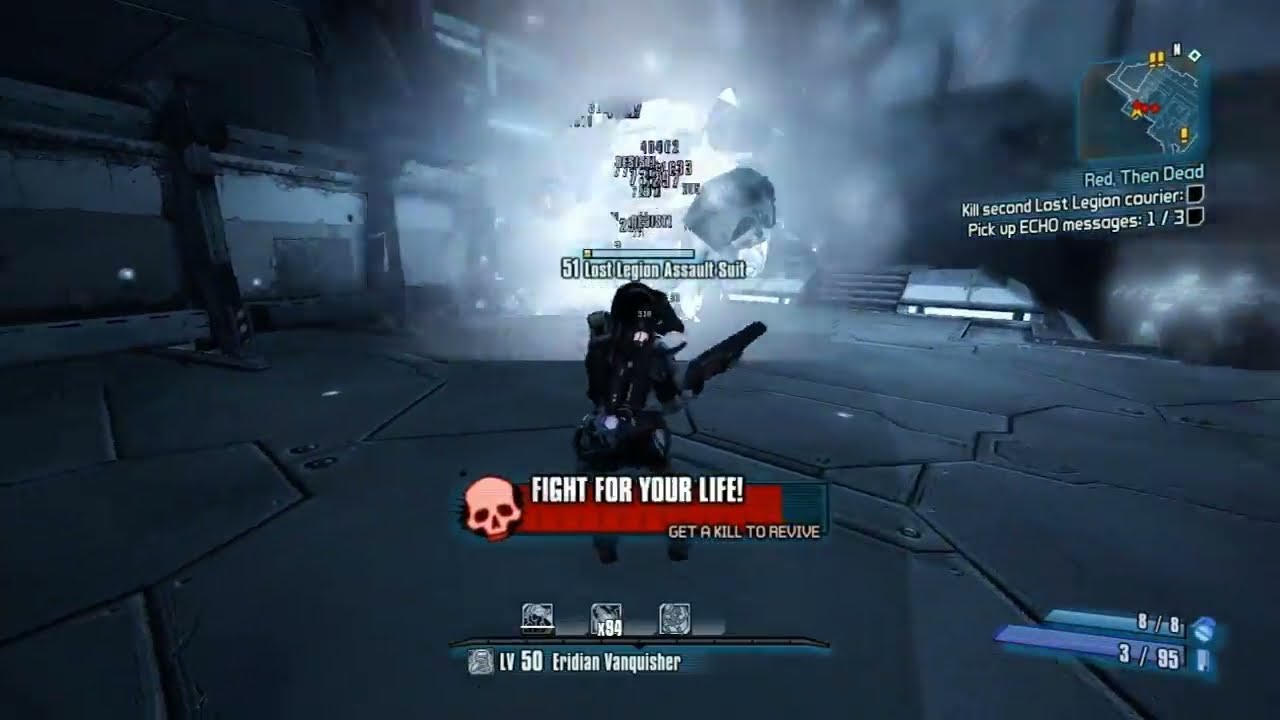The image is a highly detailed screenshot from a futuristic, hyper-realistic first-person shooter video game. The scene is dominated by a dark and blue monochromatic palette with accents of black, white, gray, silver, red, pink, and green. In the lower right corner of the screen, a gun is visibly held from the player's first-person perspective, aimed at a large, blue, monstrous figure that seems to be in the process of getting shot or exploding. This central creature appears chunky and mechanical, set against a backdrop filled with intricate, futuristic machinery and buildings.

On the upper right, game objectives are clearly displayed with the text "Kill Second Lost Legion Courier" and "Pick up ECHO messages: 1 out of 3." In the middle of the screen, large, bold letters display "LV-50 Eridian Vanquisher", possibly indicating the player's current level or status. Scattered across the screen are various point values such as 88, 49, 6,000, and 174, likely representing scores or damage indicators. Additionally, a laser beam is visible, shooting from the right to the left side of the image, enhancing the action-packed atmosphere. The overall aesthetic combines elements of realism and high-tech sci-fi, creating a visually immersive gaming experience.